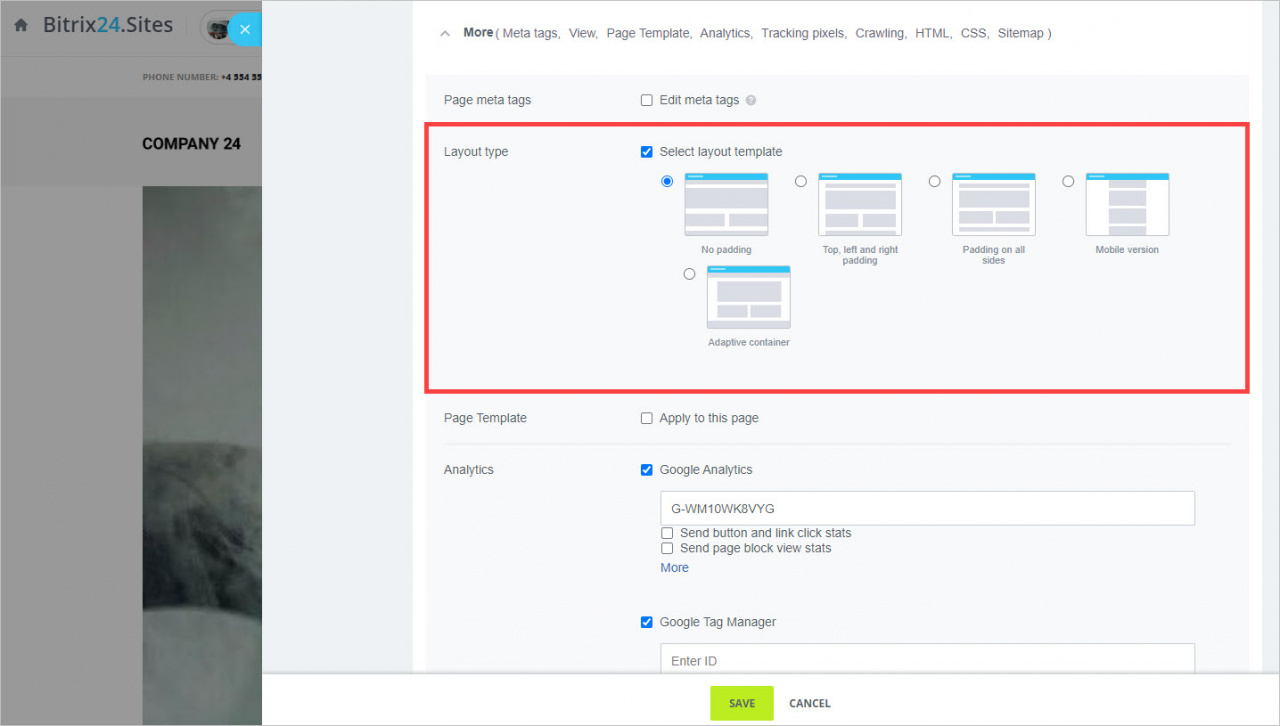The screenshot depicts a specific section of the Bitrix24.sites website, wherein a drop-down menu occupies approximately four-fifths of the image, very minimally revealing the actual webpage on the far left side, which has been grayed out. At the very top left corner, the website logo is displayed: "Bitrix24.sites" is printed, with "Bitrix" in black, "24" in blue, and ".sites" in black.

Below the logo, the text "Company 24" appears, partially obscuring a gray photo whose details are not discernible. Taking up the majority of the visible area on the screenshot, the drop-down menu has a white background and is headed by the word "More" in a gray font. It is followed by a list of options including "MetaTags," "View," "Page Template," "Analytics," "Tracking Pixels," "Crawling," "HTML," "CSS," and "Sitemap."

In a section outlined by a red rectangle, there are controls labeled "Layout Type" with the instruction to "Select Layout Template." This section showcases five mini-layout previews, each represented by small squares featuring gray blocks indicative of their respective structure. 

Below the layout selection area, the "Page Template" section appears, followed by "Analytics" and "Google Analytics" information. At the bottom of the menu, two buttons are visible: a green rectangular "Save" button on the left and a "Cancel" button on the right.